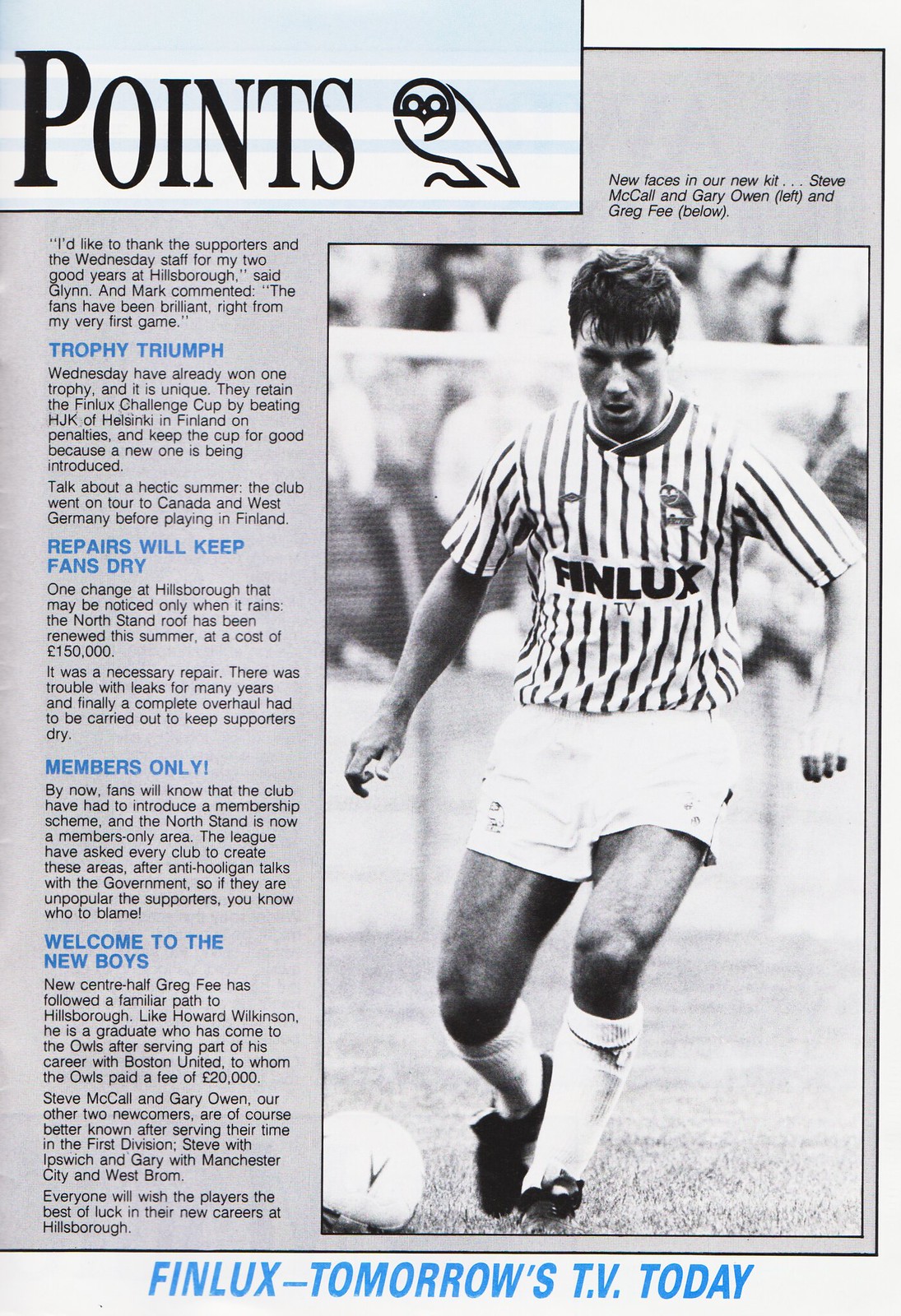This magazine page features a detailed layout with various elements. 

At the top left, there’s a small rectangle featuring blue and white stripes. Within this rectangle, the text "points" is displayed alongside a simple logo of an owl sketch. Below this rectangle, longer text appears, where the headings are written in blue and the body text in black. These headings include "Trophy Triumph," "Repairs Will Keep Fans Dry," "Members Only," and "Welcome to the New Boys."

On the right side of the page, there is a black-and-white photograph of a footballer mid-play, donning a jersey emblazoned with the same owl logo. The player is in a running position with a soccer ball on the ground in front of him. Above the photograph, text announces "New Faces in Our New Kit" featuring Steve McCall and Gary Owen on the left, and Greg Fee below.

At the bottom of the page, there’s a blue banner with the text "Finlux - Tomorrow's TV Today" against a light green background. The magazine page overall has a grayish backdrop, tying together the various sections with a cohesive look.